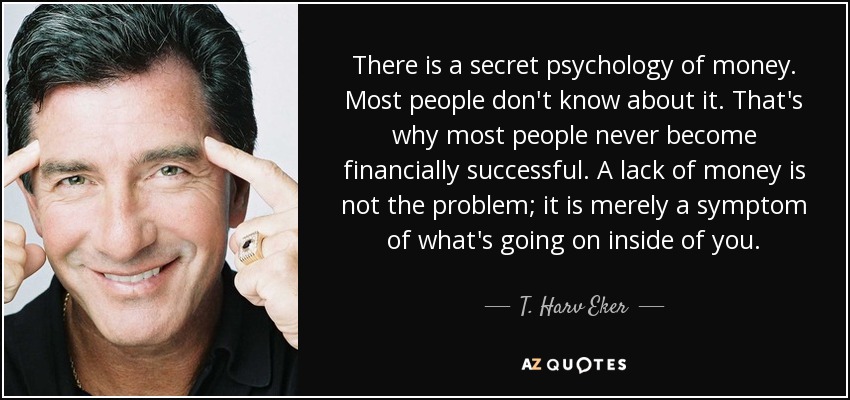The image is horizontally aligned and split into two rectangular sections. On the left side, there's a photograph of a light-skinned man with a fairly conventional and handsome appearance. He has dark hair sprinkled with a bit of gray, suggesting he might be in his 50s or 60s. He is smiling and wearing a black shirt. With both forefingers, he is pointing towards his temples, just above his eyebrows, as if deep in thought. Notably, he is also wearing a ring on his ring finger, indicating that he is possibly married. 

The right side of the image features a black background with centered white text. The text reads: "There is a secret psychology of money. Most people don't know about it. That's why most people never become financially successful. A lack of money is not the problem. It is merely a symptom of what's going on inside of you." This quote is credited to T. Harv Eker, with dash marks on either side of his name. At the bottom, the source is identified as AZ Quotes. The Z in "AZ" is orange, and the O in "Quotes" has been replaced with a thought bubble icon, resembling those found in comic strips.